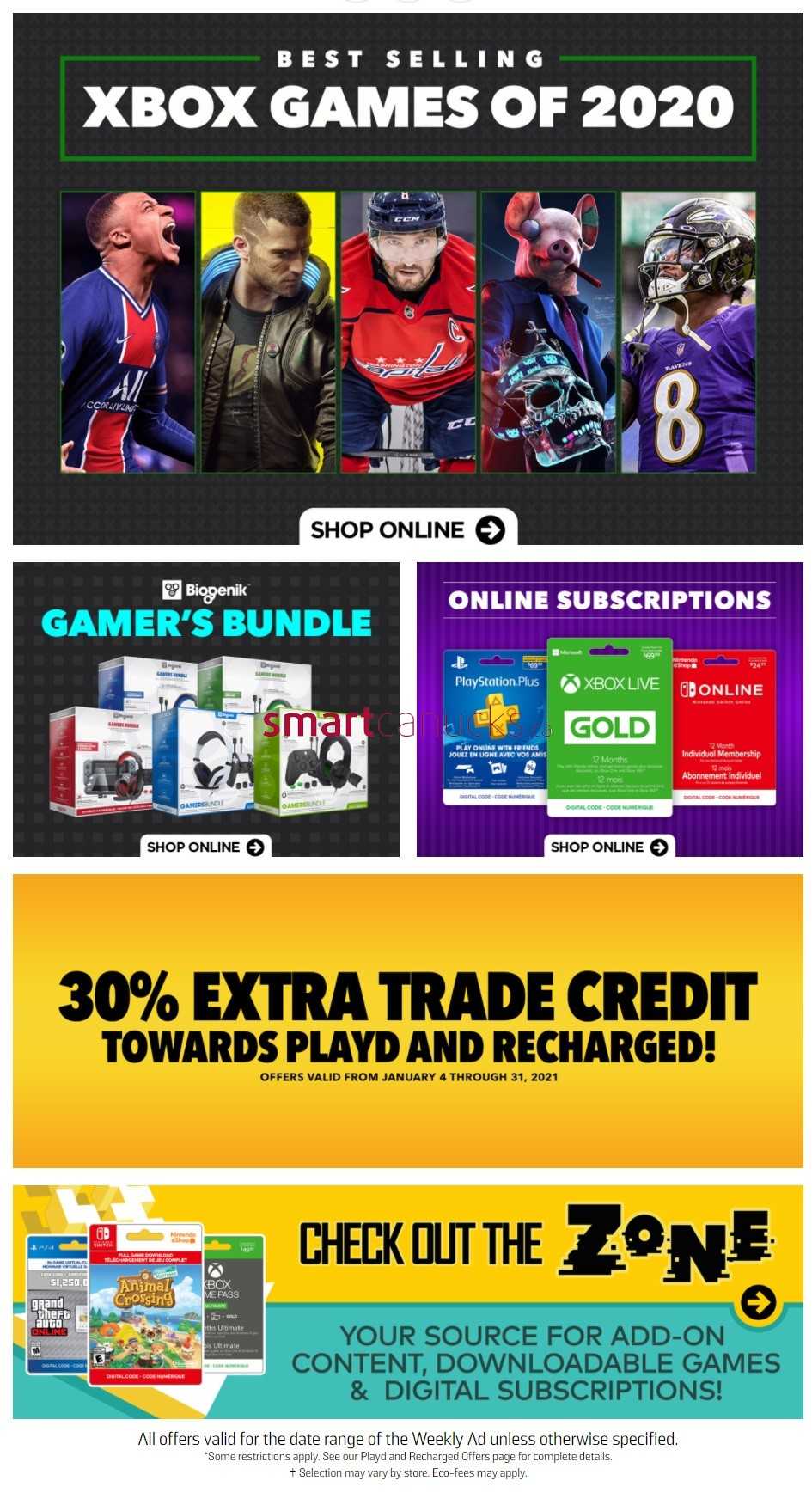The image appears to be from a promotional flyer or advertisement. At the top, the background is a dark gray with subtle lines running through it. In white letters, the header reads "Best-Selling Xbox Games of 2020". Just below this, there are thumbnail images representing various popular video games.

The lower portion of the flyer shifts to a white background with the text "Shop Online" accompanied by an arrow. Below this section, there is a gray square featuring the text "Gamer's Bundle" with images of various gaming merchandise and accessories. Adjacent to this, a purple square with white lettering promotes "Online Subscriptions," showcasing gift cards and services such as PlayStation Pro.

Further down, a yellow background with black writing announces "30% Extra Trade Credit" with the tagline "To Where It's Played and Recharged". The phrase "Check Out the Zone" adds emphasis to this offer.

At the very bottom, a blue background declares, "Your Source for Add-On Content, Downloadable Games, and Digital Subscriptions," highlighting the store's offerings for additional gaming content and digital products.